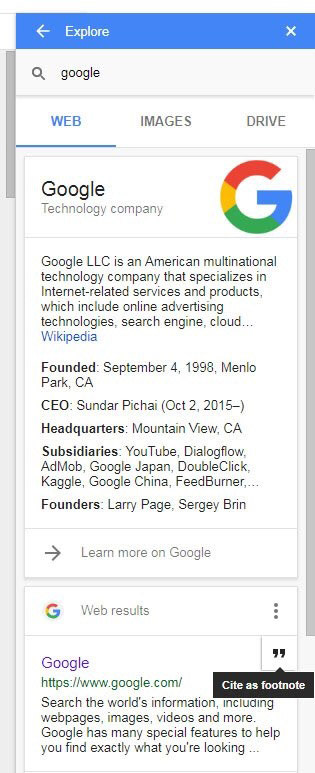This is a detailed screenshot of a mobile app interface, likely displaying search results from Google. 

At the top, there is a blue navigation bar with white text. On the left side, the word "Explore" is displayed next to a left-pointing arrow, indicating the option to navigate back. On the right side, there is a white "X" symbol for closing this section of the app or webpage.

Below the navigation bar, there is a white search bar featuring a magnifying glass icon on the left. Within the search bar, the word "Google" is displayed in gray text. 

Underneath the search bar, there are three selectable tabs labeled "Web," "Images," and "Drive." The "Web" tab is currently selected, indicated by its dark blue color and an underline.

The main content starts with a information box. On the left, it reads "Google" followed by "Technology Company." On the right of this text, there is the Google "G" logo. Below this, a brief description states, "Google LLC is an American multinational technology company that specializes in internet-related services and products, which include online advertising technologies, search engine, cloud..." trailing off with ellipsis. A blue "Wikipedia" link follows this description.

Further details include the founding date and location: "Founded: September 4, 1998, Menlo Park, California." It also states, "CEO: Sundar Pichai (October 2, 2015–)," "Headquarters: Mountain View, California," and lists some subsidiaries like YouTube, Dialogflow, AdMob, Google Japan, DoubleClick, Kaggle, Google China, and FeedBurner, followed again by ellipsis.

It also mentions the founders: "Founders: Larry Page, Sergey Brin," with a right-pointing arrow and the text "Learn more on Google." The section ends with the heading "Web results," followed by a typical Google web result format.